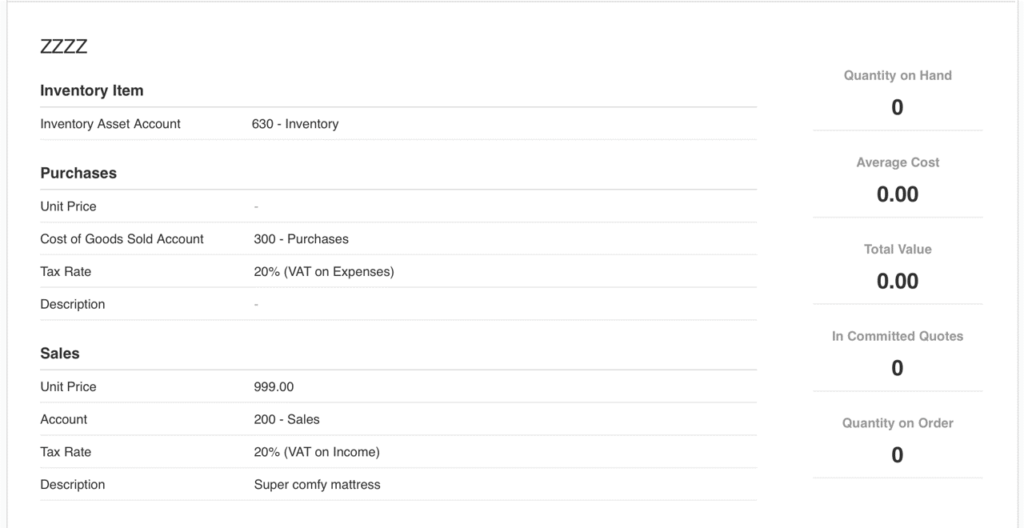This image appears to be a screenshot of an accounting or inventory management sheet with a white background and a thin gray border on the top, left, and right sides. The bottom of the image is cut off. The screenshot is horizontally oriented and contains organized textual data.

On the left side, the text begins with four 'Z's (ZZZZ), followed by bolded text that reads "Inventory Item". Just below this is a gray line dividing the sections, followed by "Inventory Asset Account" and the number "630 Inventory". This is an indication of an inventory item's classification.

The format suggests that there are two sections, one detailing inventory attributes and the other outlining financial details. Directly to the left of the "Inventory Item" section, it states "Quantity on Hand: Zero".

Below the inventory information, another section pertains to purchases and sales. Key headers in this section include "Purchases", "Unit Price", "Cost of Goods Sold Account", and "Tax Rate". The tax rate is specified as "20% VAT". 

Additionally, there is a "Description" field, and next to it on the far left, information on "Average Cost" and "Total Value" follows.

Overall, the screen appears to represent a spreadsheet or similar document used for tracking pricing, inventory quantities, and accounting details.